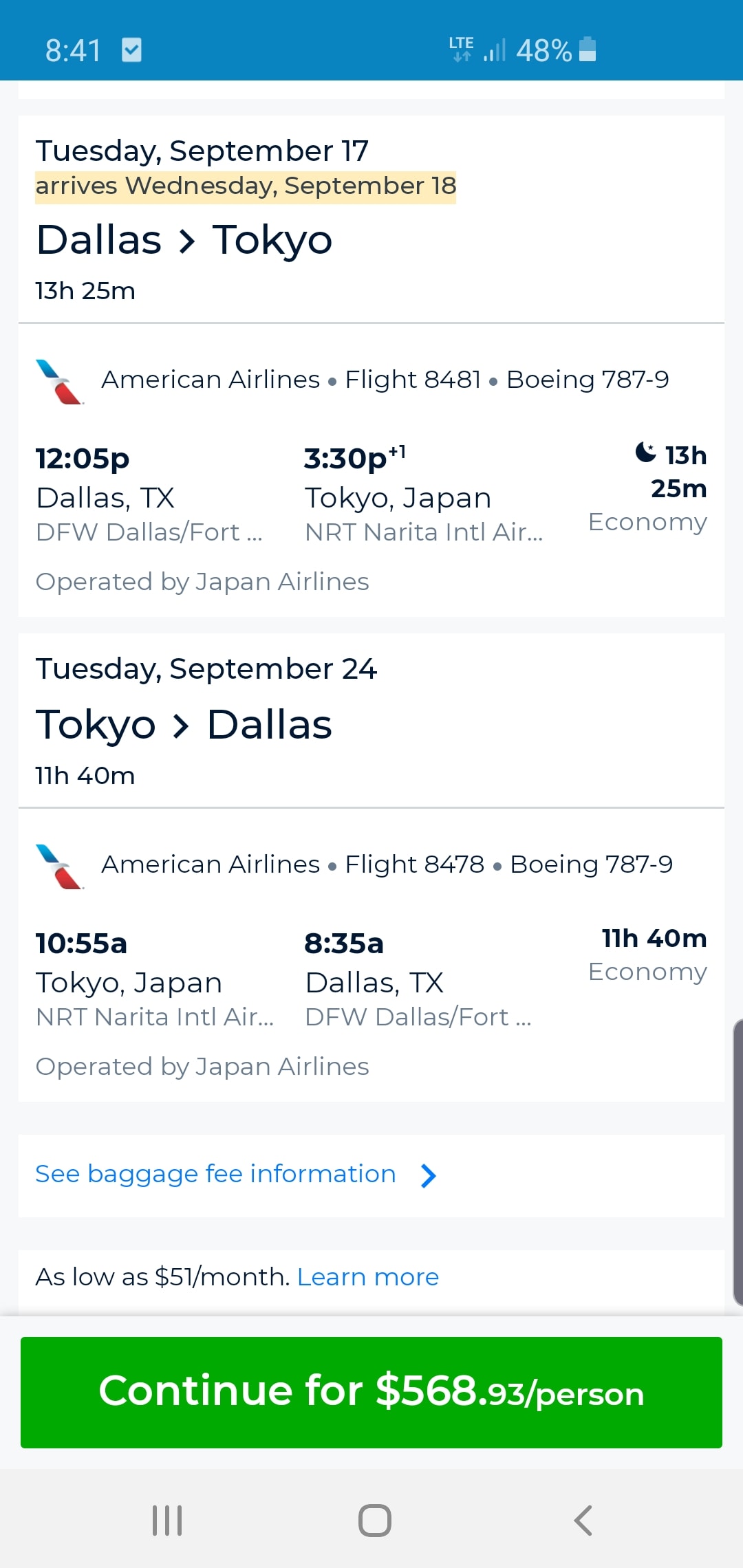**Detailed Image Caption:**

This image is a screenshot captured from an Android mobile device, evident from the presence of a navigational bar at the bottom, distinguishing it from iPhones. The content displayed is from a travel booking application or website. The interface features a predominantly white background with black text, and some elements highlighted in yellow for emphasis.

At the top, the travel dates are shown: "Tuesday, September 17th" and the arrival date "Wednesday, September 18th," both sections are highlighted in a yellowish hue. Just below, there's a route information stating "Dallas to Tokyo," with a flight duration of 13 hours and 25 minutes.

A separating line demarcates the next section, which details the flight specifics:
- Airline: American Airlines
- Flight Number: 8481
- Aircraft: Boeing 787-9
- Departure: 12:05 PM from Dallas, Texas (DFW - Dallas Fort Worth International Airport)
- Arrival: 3:30 PM (plus one day), in Tokyo, Japan (NRT - Narita International Airport)
- Duration: 13 hours and 25 minutes
- Class: Economy
- Note: Operated by Japan Airlines

Further below, the return flight information is given for "Tuesday, September 24th" from "Tokyo to Dallas":
- Flight Duration: 11 hours and 40 minutes
- Flight Number: 8478
- Aircraft: Boeing 787-9
- Departure: 10:55 AM from Tokyo, Japan (NRT - Narita International Airport)
- Arrival: 8:35 AM in Dallas, Texas (DFW - Dallas Fort Worth International Airport)
- Duration: 11 hours and 40 minutes
- Class: Economy

At the bottom of the screen, a prominent green button indicates the option to continue with booking, displaying the price of "$568.93 per person."